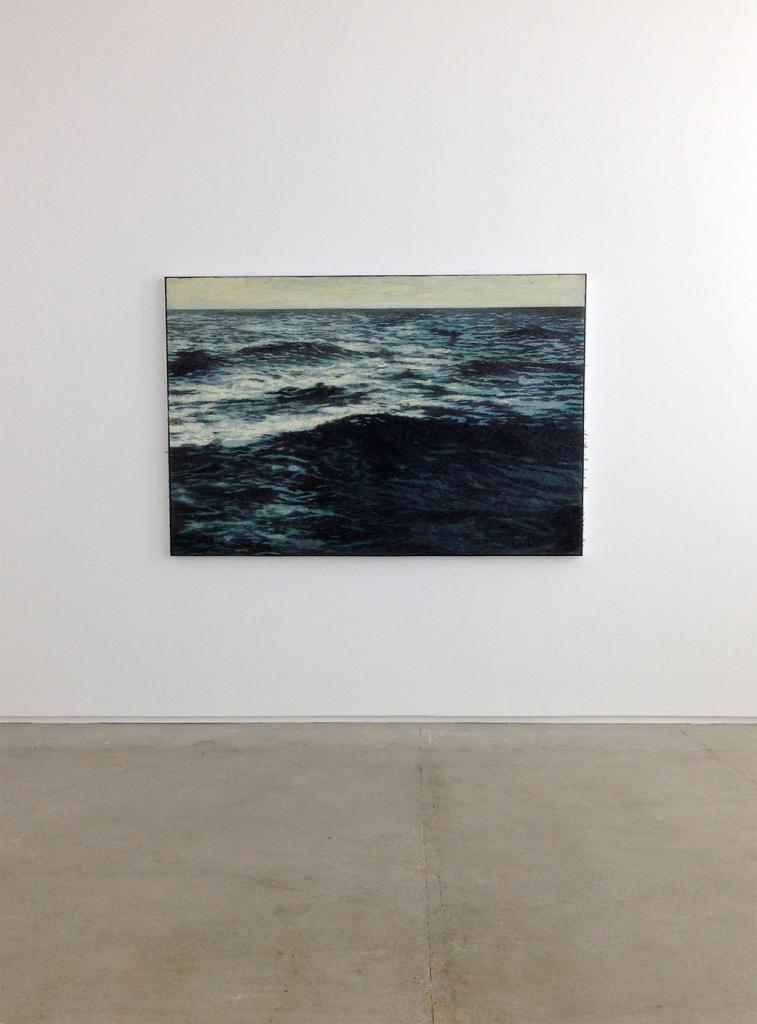The image depicts an artist's gallery with a concrete floor and a stark white wall. Hanging on the wall, relatively low, is a large rectangular photograph of the ocean. The ocean in the photograph is depicted in dark blue shades with small, non-crested waves that have black and white highlights where the light hits them. The upper part of the photograph reveals a hazy, whitish-tan horizon that contrasts with the sea, suggesting a distant horizon rather than a clear sky. The floorboard marks the transition from the concrete floor to the white wall, further enhancing the photograph's central placement. There is no text on the image, and all objects appear upright and neatly arranged.